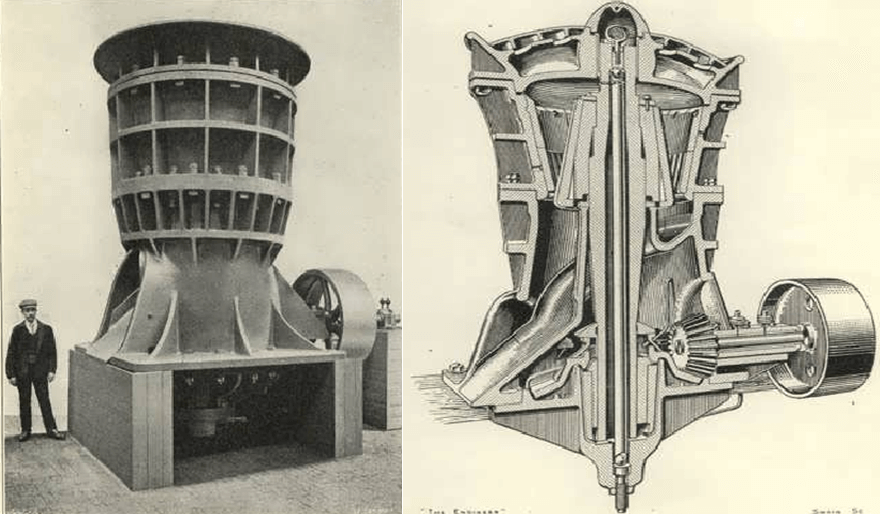The image presents a juxtaposition of a large, industrial metal machine with its intricate inner workings displayed. The composition is split down the middle, offering two perspectives: on the left, a real-life photograph of the machine, towering over a man in a suit and hat, highlighting its immense scale. The machine, cylindrical at the top and mounted on a square base, is portrayed in stark black and white tones with slight yellowish tan tints in the background. It appears to be constructed on a brick-like surface, possibly suggesting its exhibit or storage setting. On the right side of the image, there is a detailed drawing or schematic of the machine's interior, showcasing its gears, engine parts, and a central bar, revealing the complex mechanics hidden within the exterior facade. This dual representation emphasizes both the aesthetic and functional aspects of this colossal piece of engineering, potentially used in maritime or industrial applications.